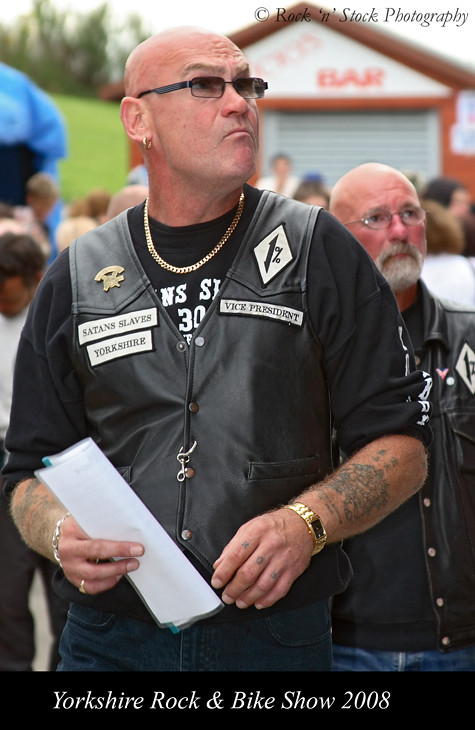The image, taken in an outdoor setting and labeled with the text "Rock and Roll Stock Photography" in the top right corner, prominently features two bikers at the Yorkshire Rock and Bike Show 2008. At the forefront, a man with a shaved head, wearing black sunglasses and a gold hoop earring, is dressed in a biker vest over a black T-shirt adorned with gold necklaces. His vest bears the insignia "Satan Slaves, Yorkshire Vice President" on the left and right sides respectively. He has tattoos covering both arms and across his knuckles, although the knuckle tattoos are not readable. A watch on his left wrist and a bracelet along with a ring on his right hand are noticeable. He is holding a folded white paper with a slide sleeve front. Dressed in dark jeans, he stands in front of a shop front with a grey sky and blurred grass and trees in the background.

Next to him is another man, similarly attired with a shaved head and glasses. This man has a white beard and is also dressed in biker gear, but wears a jacket instead of a vest. The background also includes other people, emphasizing the communal atmosphere of the event. At the bottom, a banner clearly states "Yorkshire Rock and Bike Show 2008" in white writing.